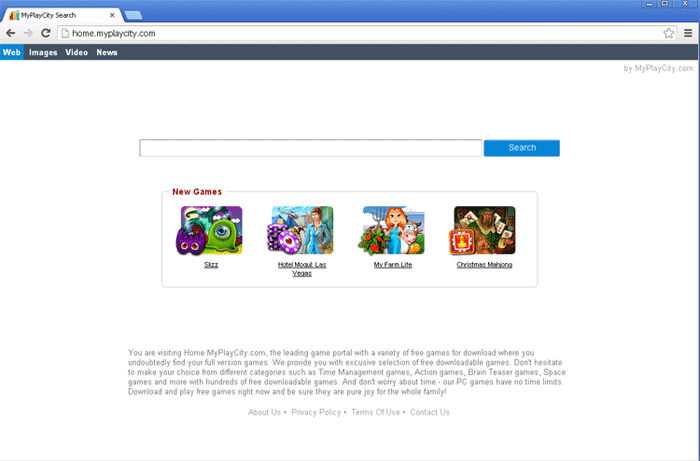This rectangular image, oriented horizontally from left to right, depicts a web browser interface centered on a search page titled "MyPlayCity Search." The top section features standard browser navigation tools, including a left-pointing arrow, a semicircular refresh icon, and an "X" to close the page. Displayed next to these tools is the URL "home.myplaycity.com." Toward the right side of this bar, familiar Windows icons are present: a star for bookmarking, a dash for minimizing, a square for maximizing, and another "X" for closing the window. Additionally, a hamburger menu icon is positioned on the far right.

Below this initial section, there is a black border serving as a separator, containing the menu options "Web," "Images," "Video," and "News," all rendered in white text. The "Web" tab is selected, indicated by its blue highlight. In the next section, a white search field with a blue search button to its immediate right invites user interaction.

Further down, the page features a section labeled "New Games." Within this area, there are four smaller boxes each showcasing a thumbnail of new games available. While the details of all the games are not entirely clear, the titles of the second, third, and fourth games are visible: "Hotel Mogul Las Vegas," "My Farm Life," and "Christmas Making," respectively.